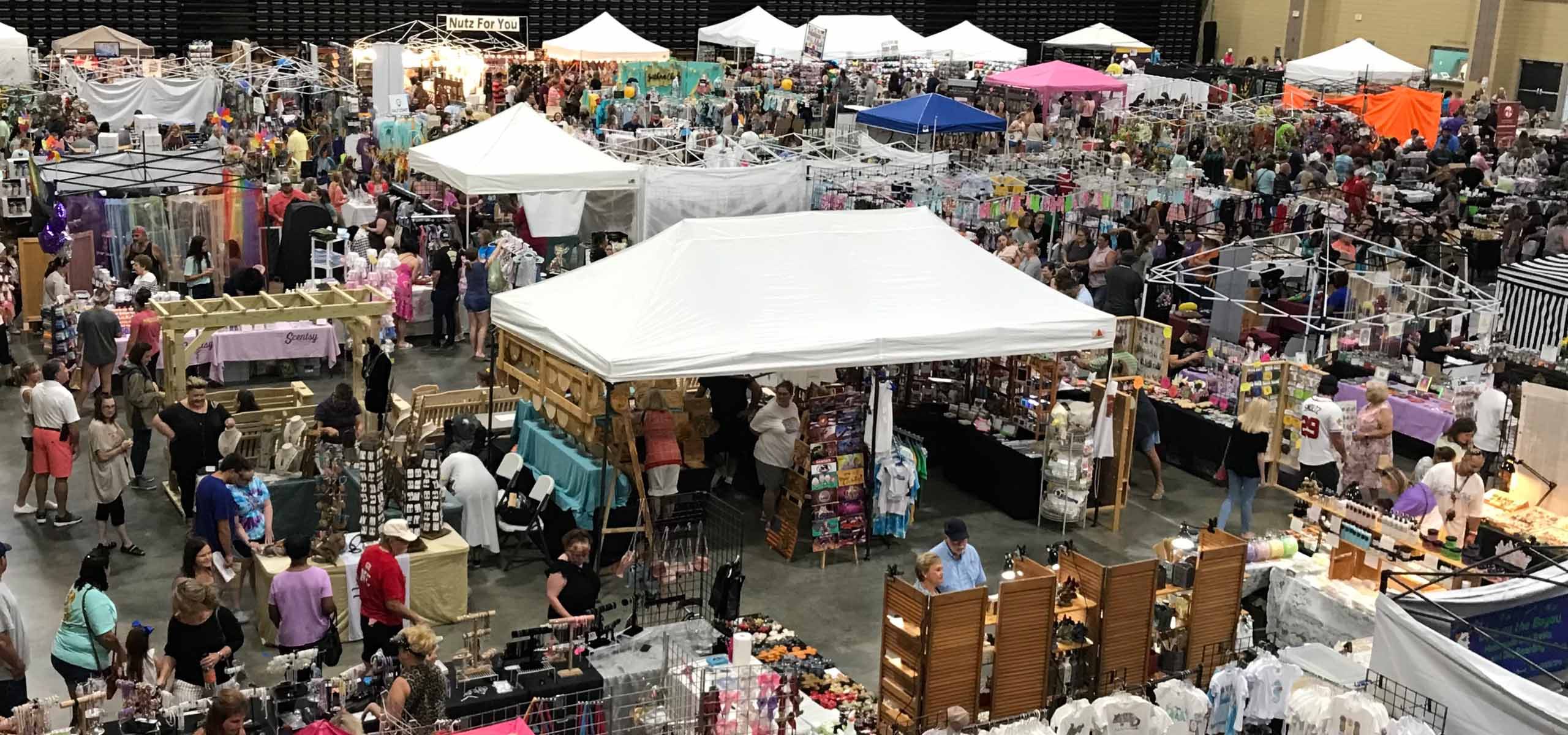In this indoor flea market or craft show, we see an array of colorful stalls and bustling activity. The backdrop is defined by brown and black walls, with a reflective cement-gray floor adding to the indoor ambiance. Multiple tent covers, predominantly white, are interspersed with a few blue, pink, and an orange one, which appears torn. The market features a variety of colors from participants' clothing, including teals, blacks, purples, reds, and greens. Notably, in the bottom left, a man in a gray t-shirt and face cap stands next to a woman in a green t-shirt. On the left side of the image, there’s a signboard reading "NUTZ for you." Various wooden display stands, possibly selling handcrafted wooden items, are noticeable, especially on the bottom right. The scene is a lively indoor environment where vendors display their products to interested consumers.